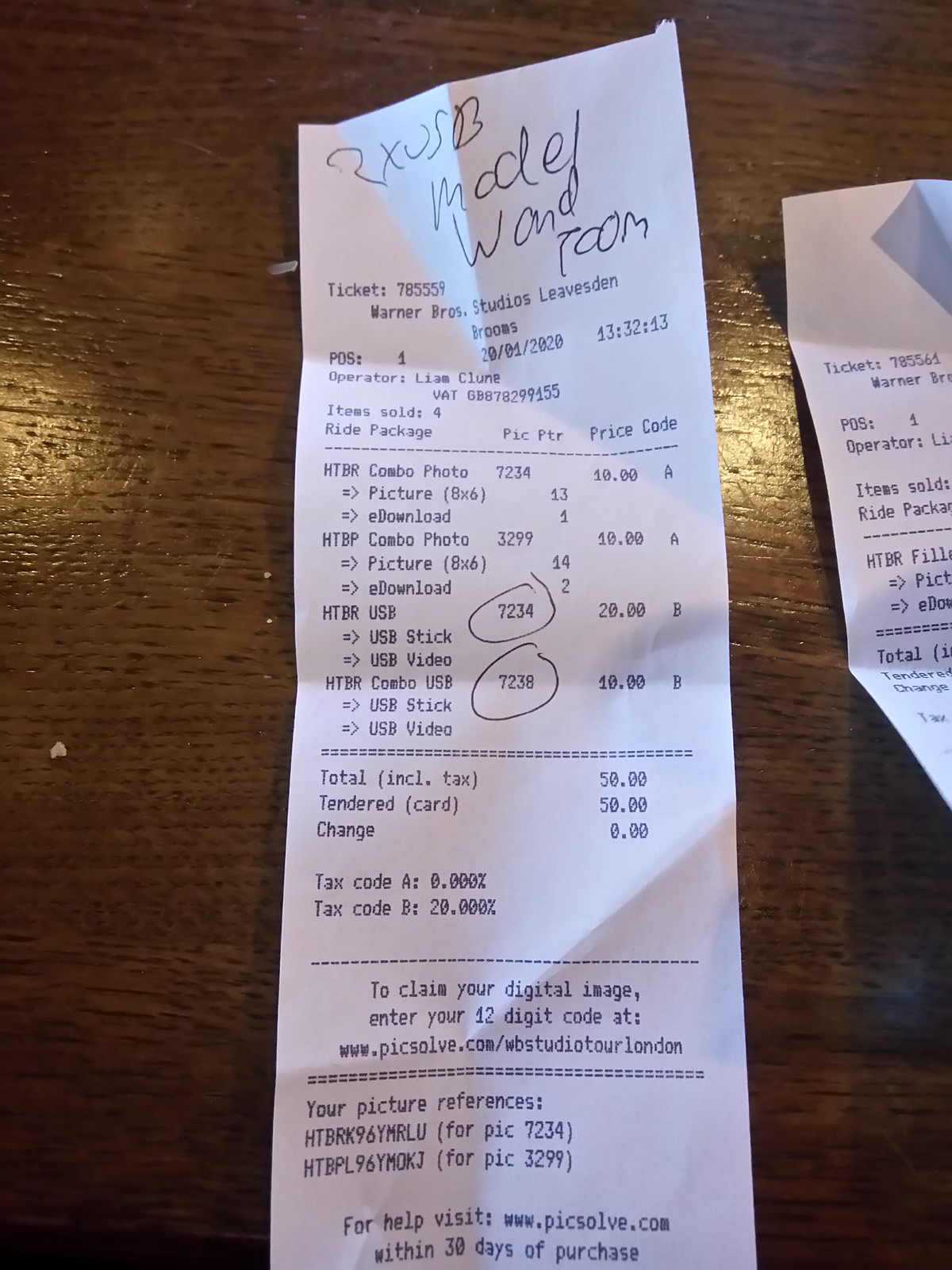This detailed portrait-style image captures a receipt laid out on a brown wooden table. The white receipt, adorned with black text, reads "Warner Bros. Studios Leaves Den. Brooms Operator Liam Clune, 20-01-2020, 13:32:13." The main purchase items listed are "HTBR Combo Photo $10 picture and e-download," "HTBR USB $20," and "HTBR Combo USB $10," summing up to a total of $50. The transaction was completed with a card payment of $50, leaving $0 in change. Intricate details include small, handwritten numbers and letters at the top of the receipt, indicating something like "2X0SB model wand foam or zoom," and a ticket number "785559." To the right is a partial view of another smaller white receipt, making up approximately 30% of it as it's cut off at the edge of the image. The table’s dark brown surface is slightly irregular with a tiny white crumb visible on the left-hand side, adding a touch of realism to the scene.